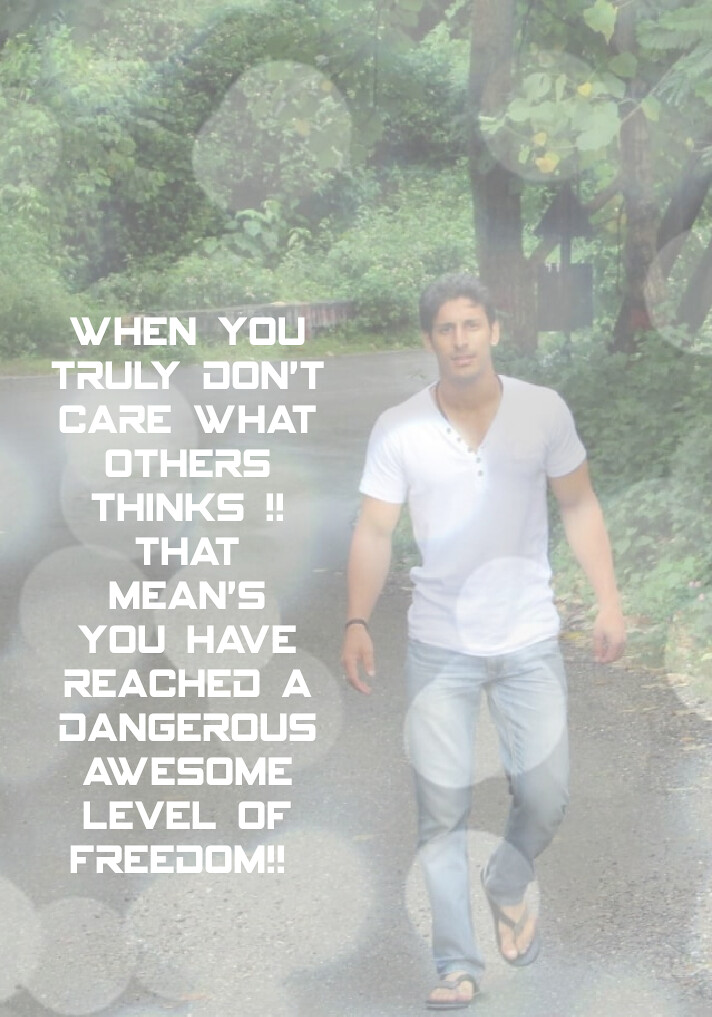The image displays a somewhat faded and blurry outdoor scene featuring a man walking along a pathway. He is dressed in blue jeans, sandals, and a light-colored or white t-shirt, and appears to be wearing a bracelet on his right arm. The pathway is marked with a gray design that includes lighter gray circles. To his left, a striking quote in white, all caps text reads, "WHEN YOU TRULY DON'T CARE WHAT OTHERS THINK, THAT MEANS YOU HAVE REACHED A DANGEROUS AWESOME LEVEL OF FREEDOM!" The background includes a considerable amount of greenery—grassy areas, numerous trees, bushes, and a faintly visible fence. Above the man's right shoulder, a dark, indistinct street sign with a triangular shape is present. The overall image has a milky film and patches of discoloration, contributing to its faded, textured appearance.